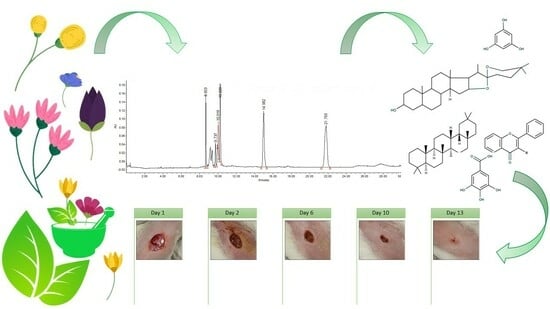The image is a detailed diagram explaining the growth cycle of a flower from seed to blossom. The timeline is marked with specific days: Day 1, Day 2, Day 6, Day 10, and Day 13, highlighting key stages of the plant’s development. The bottom section of the diagram displays images of the seed's progression over these days. To the right of the timeline, a green arrow charts the increasing height of the growing plant, with measurements indicated at various points. 

Accompanying the timeline, the left side of the diagram features illustrations of different flowers and leaves, including three pink flowers, one blue flower, two yellow flowers, one purple flower, two more yellow and red flowers, and two green leaves, some of which are situated in a green pot. Additionally, octagonal symbols and another green arrow emphasize the continued growth of the seed, which is depicted in red.

The diagram also includes a chart tracking the changes in chemical input over time, showing both spikes and drops in chemical levels corresponding to different days. This visual representation provides a comprehensive overview of the stages of the plant’s growth, supported by colorful illustrations and detailed graphical data.